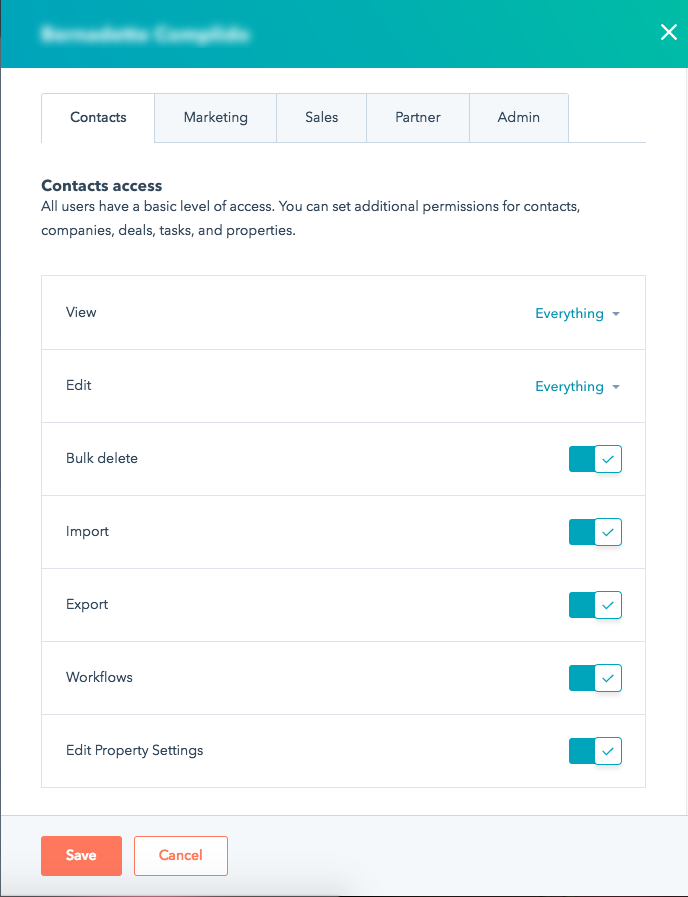### Detailed Descriptive Caption:

The image is a screenshot of a software interface window situated in the upper left corner of a screen. The top portion of the window features white text that has been intentionally blurred out and is unreadable. In the upper right corner, there is a white 'X' icon for closing the window.

Directly below the top bar, a horizontal menu is presented. The first item on the left is labeled "Contacts" and is highlighted, indicating it is currently selected. The subsequent menu items include "Marketing," "Sales," "Partner," and "Admin," aligned from left to right.

Underneath the horizontal menu, a section titled "Contacts Access" is visible. This section explains that all users have a basic level of access, and it is possible to set additional permissions for contacts, companies, deals, tasks, and properties. 

Along the left side of this section, a vertical list of options is outlined. These options include "View," "Edit," "Bulk," "Delete," "Import," "Export," "Workflows," "Edit," and "Property Settings." 

At the bottom of the window, there are two buttons: an orange button, whose specific label is not provided, and a white "Cancel" button next to it. The layout and design elements imply a user interface for managing contact information and permissions within a software application.